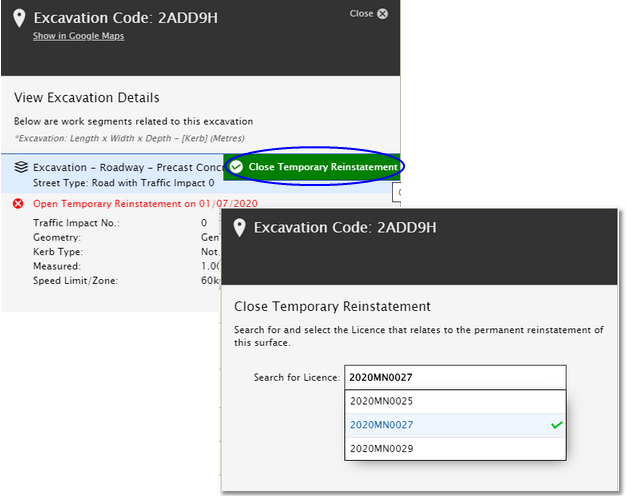A detailed screenshot displays two sections of an excavation interface. In the upper left section, a large black banner with white text reads "Excavation Code 2ADD9H." The top right corner features a "Close" button, highlighted in white text with an 'X'. Directly below, there's an option to "Show in Google Maps." Further down, a black text line indicates "View excavation details." This is followed by a segment titled "Work segments related to this excavation," detailing the excavation's dimensions (length x width x depth) and listing curb meters. A light blue banner beneath it reads, "Excavation, Roadway, Precast, Street Type, Road with Traffic Impact 0," in black text. In red text, it states "Open Temporary Reinstatement on 1-7-2020, Traffic Impact Number 0."

In the lower right section, another black banner displays "Excavation Code 2ADD9H." Below this, on a white background, black text indicates "Close Temporary Reinstatement." The structured layout and multiple banners provide a clear view of the excavation's status and related actions.